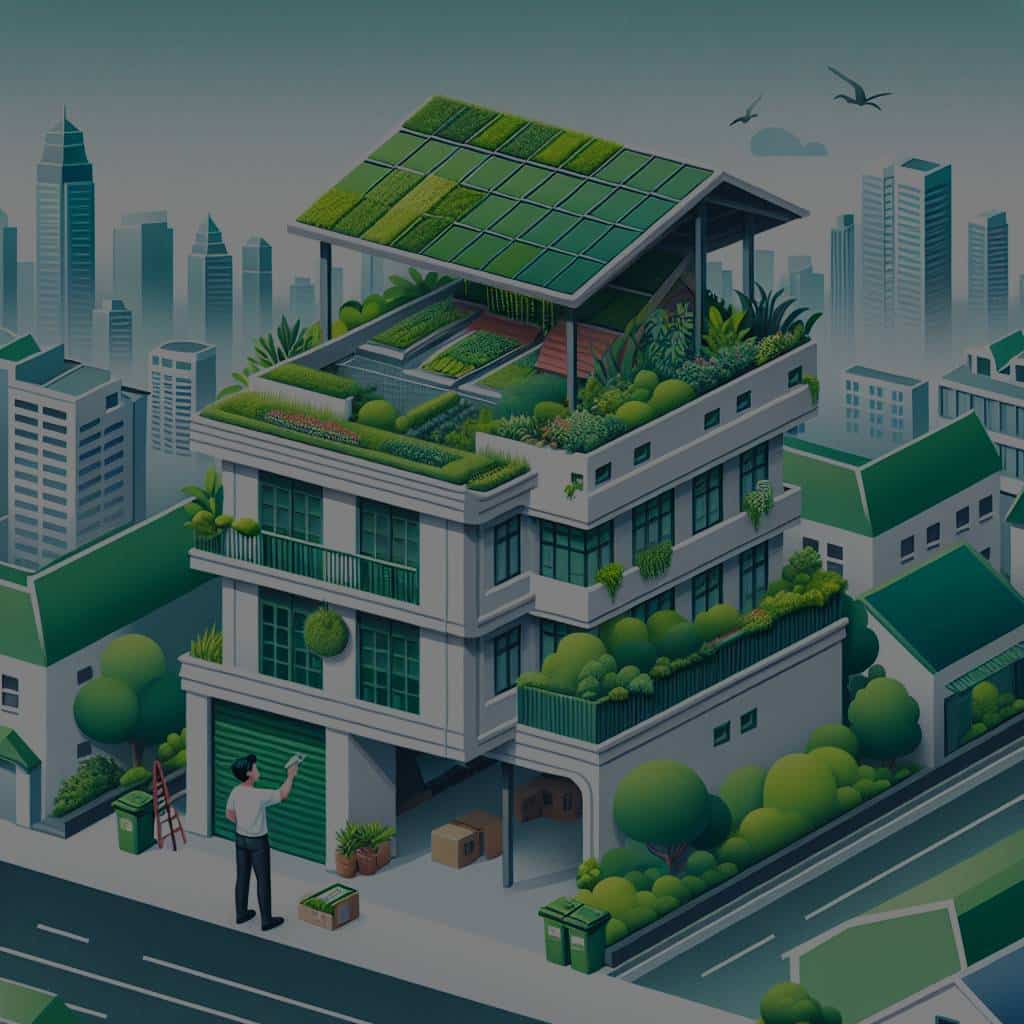This daytime, cartoon-style drawing depicts a man standing in front of a three-story house with a detailed and vibrant exterior. The house, which appears to be a mix of white and gray, features a drive-in garage on the lower level where the man with his arm raised is painting the garage door. To the right of the house, a road runs parallel, while the left side of the scene is dominated by a city skyline, with several skyscrapers veiled in a light haze and clouds, and two birds visible in the sky. 

The architecture of the house is quite intricate: the front section is a rectangular form, while behind it, another square tower rises. There is a balcony on the right side of the house adorned with numerous trees. The top of the third story supports a roof garden flourishing with abundant trees and plants. Above this garden sits another structure capped with a gabled roof, on which solar panels, covered partially in green grass, are installed. 

In addition to the main house, there's a smaller green house with a gabled roof positioned behind it. The overall scene blends urban and natural elements seamlessly, with plenty of greenery integrated throughout the architecture, giving a refreshing contrast to the nearby cityscape.